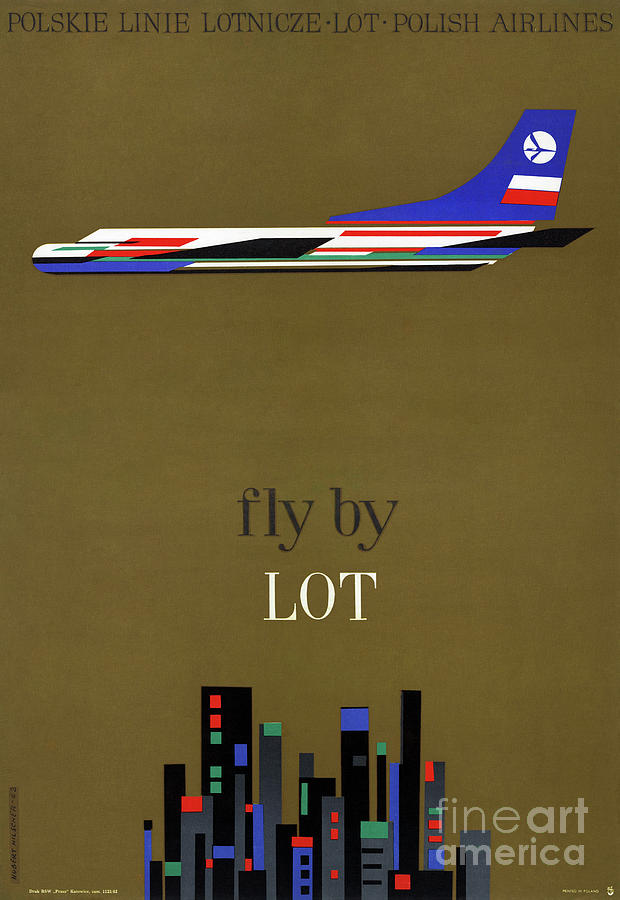This detailed artwork, resembling an advertisement, features a sleek, side-view plane set against a rich brown background. At the top, bold black lettering stretches from left to right, reading "Polski, Lanai, Laniczi, LOT, Polish Airlines." Just below this, nearly spanning the width of the vertical frame, is the sleek airplane, primarily white with red stripes. The plane's tail is blue, adorned with a circular logo and a white and red stripe beneath it. Centrally positioned text reads "fly by" in black, followed by "LOT" in white. Below this, a simplified cityscape emerges, populated with variously colored tall buildings, predominantly in blacks, grays, and blues. The windows of these buildings are highlighted with red and green accents. In the bottom right corner, a watermark reads "Fine Art America."